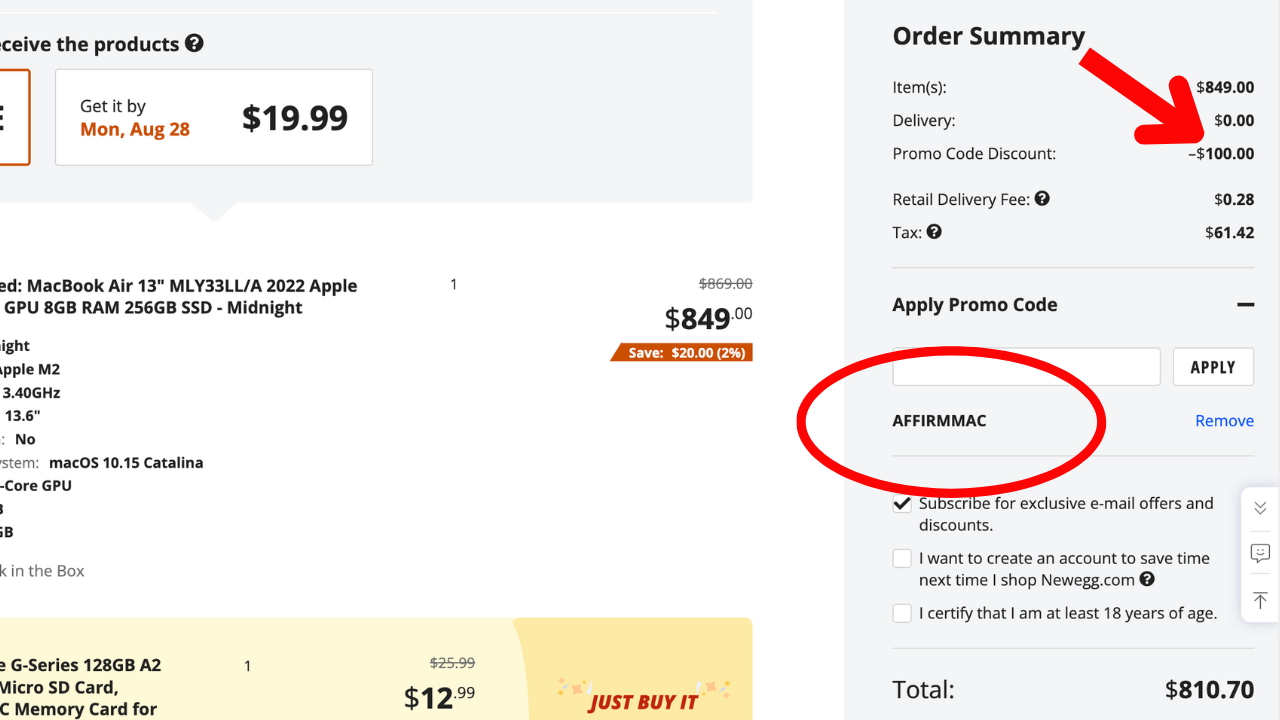This image is a detailed screenshot of an e-commerce website displaying a product page and an order summary. On the left side of the page, there is a white-based background accented with yellow, orange, and black text. The focal product is a MacBook Air 13-inch (2022) with an Apple GPU, 8GB RAM, and a 256GB SSD, available in a midnight color. The price is listed as $849, reflecting a savings of $20 or 2%. There is a sidebar offering an additional add-on item: a micro SD card for $12.99. A prominent circle button with a question mark and a delivery note stating, "Get it by Monday, August 28th for $19.99," are visible. The caption provides a detailed view of the "Just Buy It" button, which features a gradient of light to dark yellow. On the right side of the screenshot, the order summary lists the MacBook Air at $849, with free delivery, a promo code discount of $100, and tax amounting to $61.42. The grand total for the order is calculated to be $810.70.